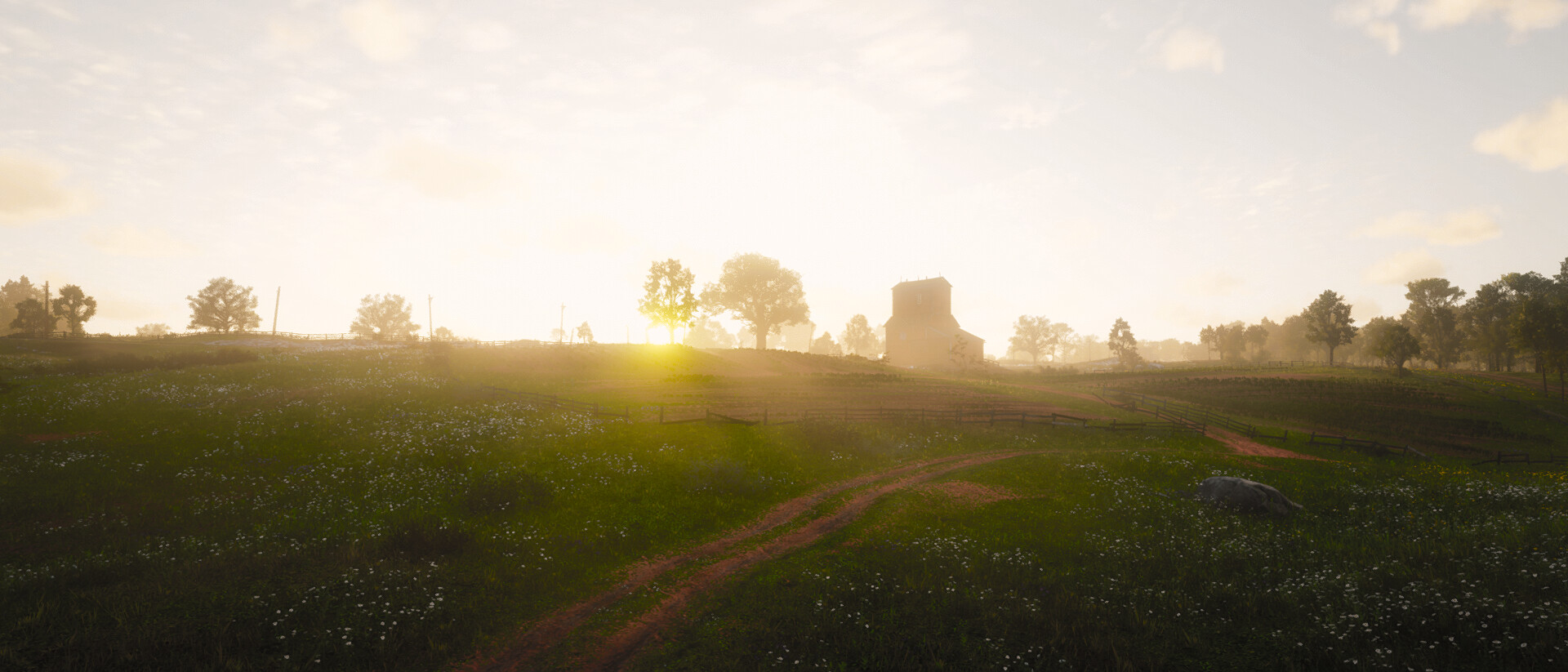This panoramic, wide-angle photograph captures a serene countryside scene during the early morning hours. The composition, which is three times as wide as it is tall, features a one-lane dirt road winding up a gently sloping hillside. Silhouetted against the light blue sky, accented by a few fluffy white clouds, stand several individual trees. The morning sun sits low on the horizon, casting a golden glow and long shadows across the landscape. At the summit of the hill, an intriguing silhouette of an old, mine-like building with an elevator tower is visible, adding a historical and mysterious element to the scene. Both sides of the dirt road are bordered by fields covered in grass and patches of clover, which lend a lush, green contrast to the earthy tones of the path. Overall, the image conveys a tranquil and picturesque rural environment at the break of dawn.